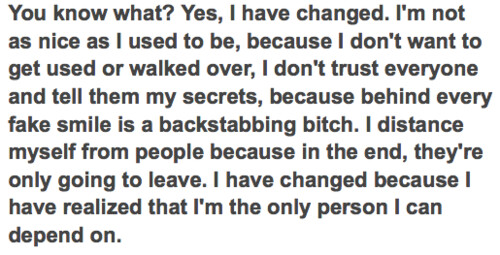In this provocative and evocative image, we see a meticulously laid out text in black on a stark white background. The quote reads: "You know what? Yes, I have changed. I'm not as nice as I used to be because I don't want to get used or walked over. I don't trust everyone and tell them my secrets because behind every fake smile is a backstabbing bitch. I distance myself from people because in the end they're only going to leave. I have changed because I have realized that I'm the only person I can depend on." The straightforward, thought-provoking text captures raw, personal reflections on self-reliance and the guarded nature that comes from past betrayals. The simplicity of its presentation, reminiscent of classic MySpace quotes, adds a nostalgic yet timeless quality, making the image both relatable and strikingly honest. The lack of additional context invites the viewer to delve deeper into its emotional resonance, casting the words as a poignant declaration of independence and self-protection.